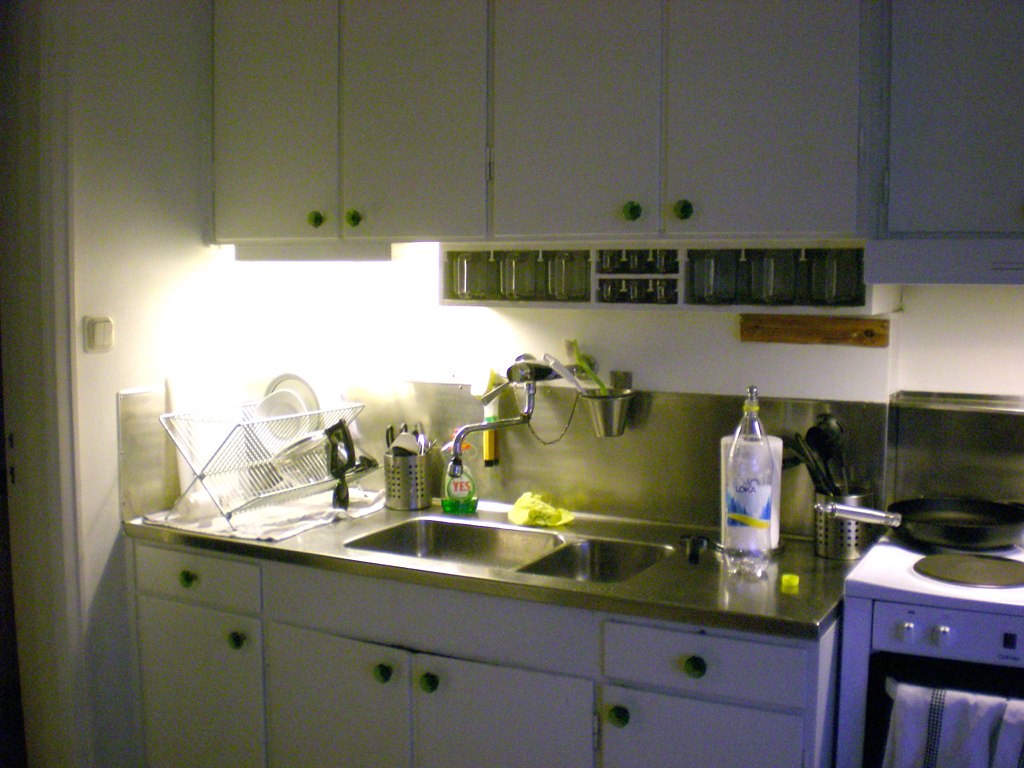The image depicts a simple yet functional kitchen. In the foreground, we see a double-bowl sink embedded in a white worktop, with a large, adjustable tap that can be directed into either sink bowl. Below the worktop, there is a white cabinet featuring four doors and two drawers for storage. To the left of the sink, a dish drying rack is neatly placed, while above the sink hangs a matching set of overhead cupboards, illuminated by an under-cabinet light. Flanking the sink are two metal cylinders filled with various kitchen utensils like knives and ladles.

The countertop also hosts a roll of kitchen paper and a plastic bottle, once containing a soft drink, now without its yellow lid. On the right side of the sink, an old-style white electric cooker with black hobs stands. A black frying pan with a silver handle rests on one of the hobs, and a dish towel hangs over the oven's door, drying. Just to the left in the image, there's a door leading out of the kitchen with a large light switch positioned next to it. The overall lighting and arrangement create a practical and cozy kitchen atmosphere.